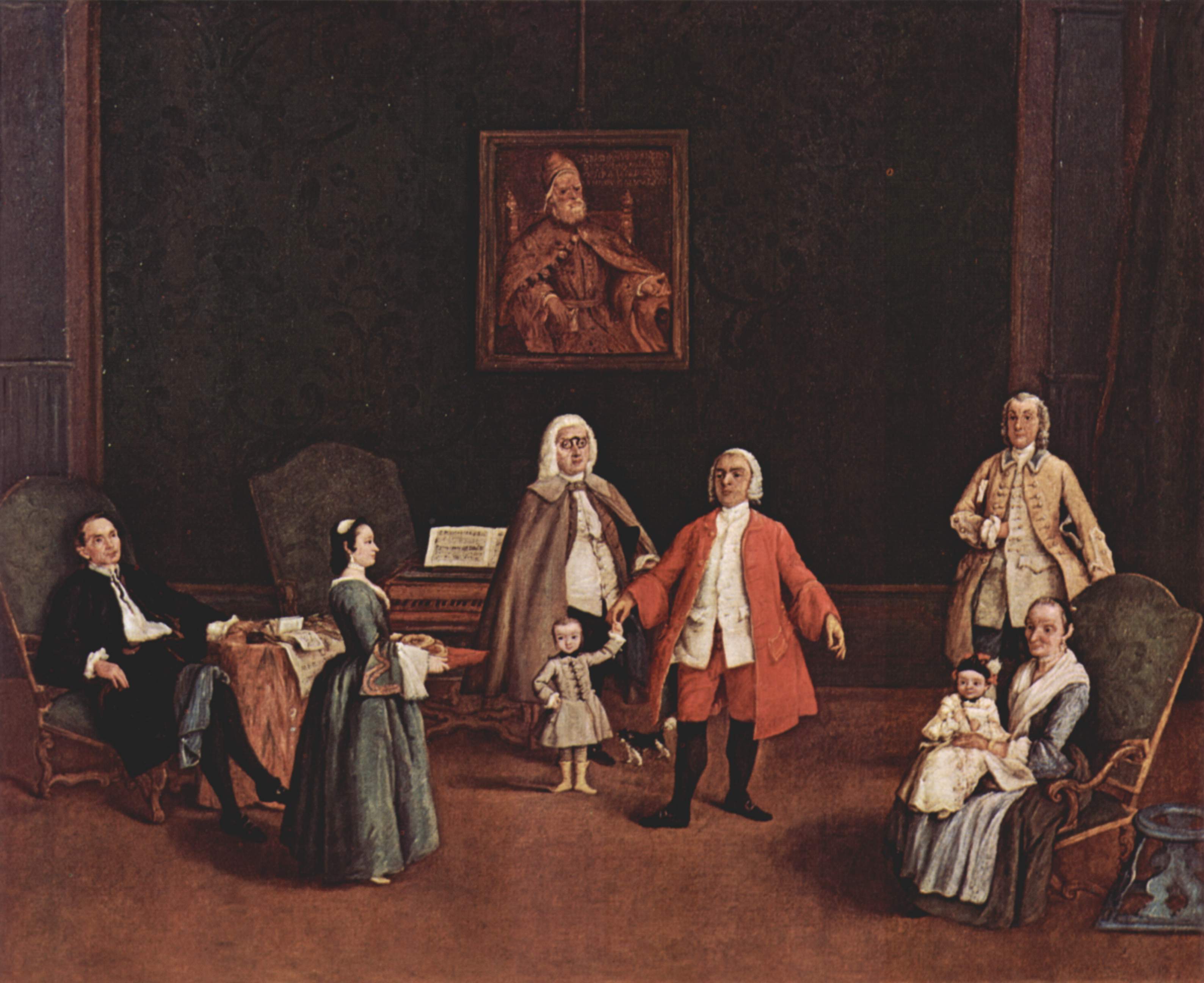This wide rectangular painting captures the interior of a grand room with dark mauve walls featuring black floral designs. Dominating the top center of the composition is a framed portrait of a solemn man with a white beard, seated on a throne and adorned in ornate brown robes and a headpiece, suggesting a figure of religious or authoritative significance.

Below, the scene is populated by eight figures dressed in 18th-century attire, arranged across a reddish-gray floor. Central to the arrangement is a small child, confidently standing in a dress-like garment and light yellow boots, holding the hand of a man in a powdered wig, red jacket, and knee-high black boots. Adjacent to them stands another man in a long brown cloak, also wearing a powdered wig.

To the left, a woman in a very dark blue dress with a bustle stands, possibly a servant, holding a plate of food and gazing towards the center. Seated nearby in one of the two large chairs is a man with dark hair, pale complexion, and a dark jacket, his attire completed by a white shirt with intricate cuffs and collar and a thin brown tie. On the far right, an elderly woman sits in a chair holding a baby on her lap, with another older man standing behind her, wearing a tan coat. The puritanical atmosphere is further accentuated by the subdued, earthy tones and the formal, almost solemn demeanor of the figures.